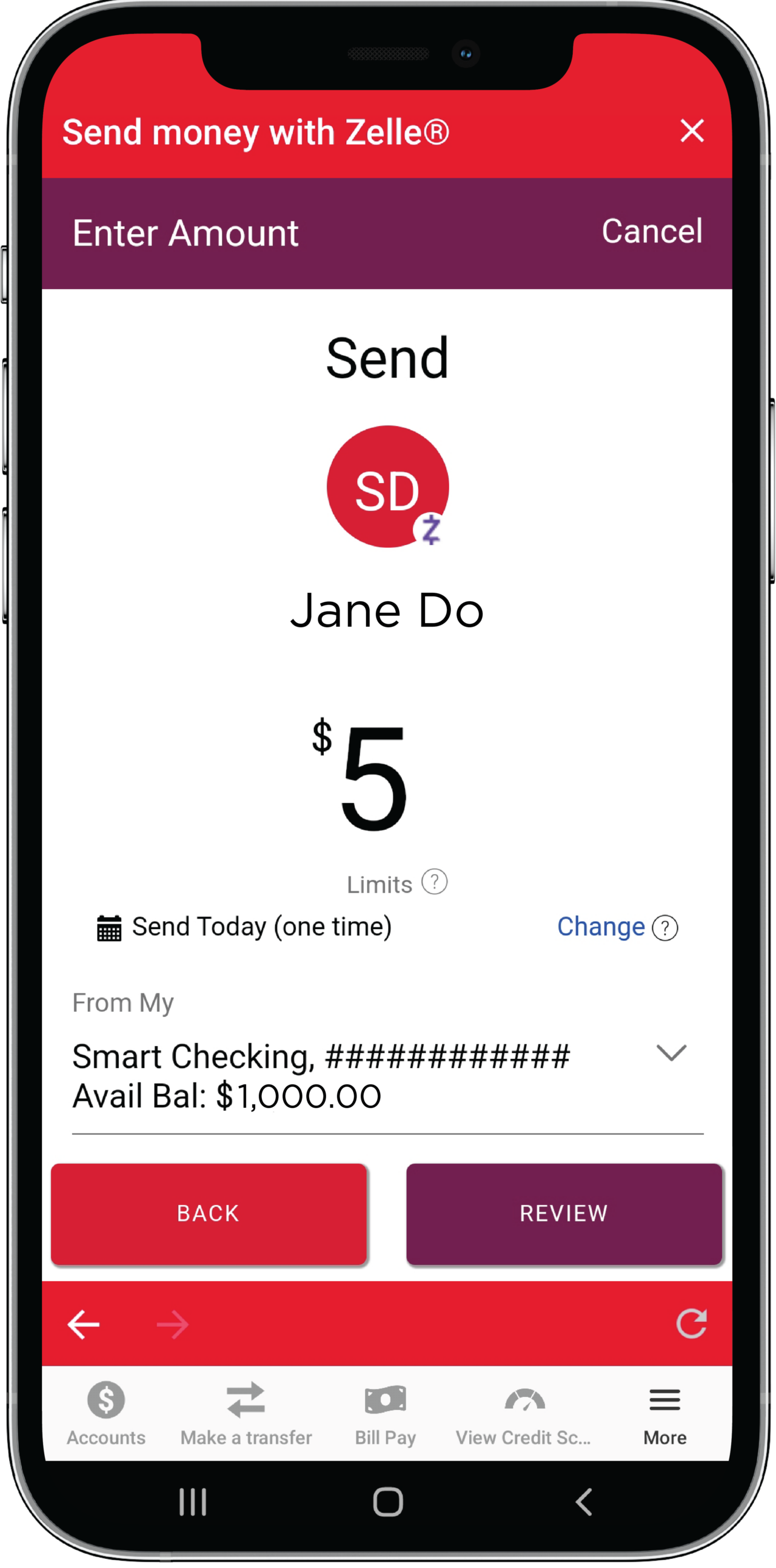Set against a stark white background, the image features a sleek black cell phone. The left side of the device has three buttons: two regular buttons and a smaller silver button above them. On the right side, a single button is visible. The phone's screen is lit, displaying a red header at the top with the white text reading, "Send money with Zelle."

Below the header is a purple banner with white text, instructing "Enter amount" on the left and offering a "Cancel" option on the right. The main part of the screen has a white background with a central black text reading "Send." Underneath, there is a round red circle containing the white letters "SD." Just below this, the name "Jane Doe" is displayed, accompanied by the amount "$5."

Further down, there’s a calendar icon with the text "Send today one time" next to it, and to the right, a blue hyperlink labeled "Change." At the bottom of the screen, there is a financial note that reads, "From my smart checking, available balance $1,000."